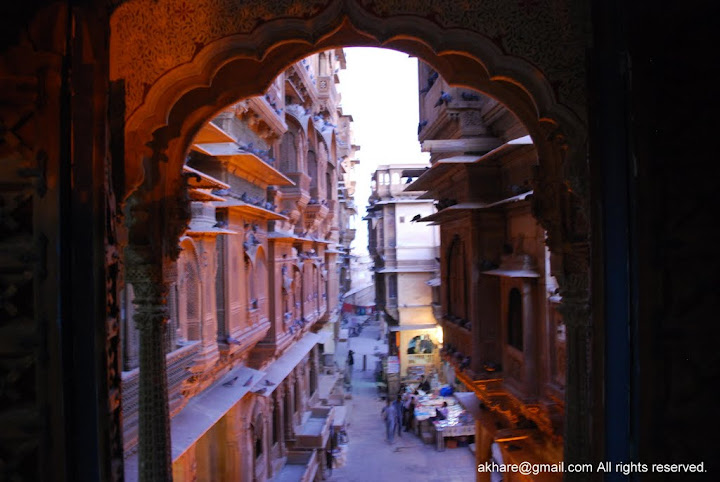The photograph captures a vibrant outdoor street scene, framed by an ornately designed, stone archway with a Moroccan-style fluted curve. The image is taken from the inside, looking out towards a narrow alley or small street that meanders through what appears to be a possibly European city. The archway itself is shadowy, with a faint reddish-brown hue on its left side. 

Beyond the arch, tall buildings, six to seven stories high, with stone facades line both sides of the narrow street, which is bustling with activity. Various market carts and tables filled with items for sale line the street, drawing a crowd of people milling about, engaging in buying and selling. Some of the buildings exhibit signs of ongoing repairs, adding a touch of the ancient charm. 

The scene is illuminated by a yellowish light source slightly to the right in the center, contrasting with the white, hazy daytime sky that forms the backdrop. At the very bottom right of the image, the text reads "akhare at gmail.com. All rights reserved" in blue font.